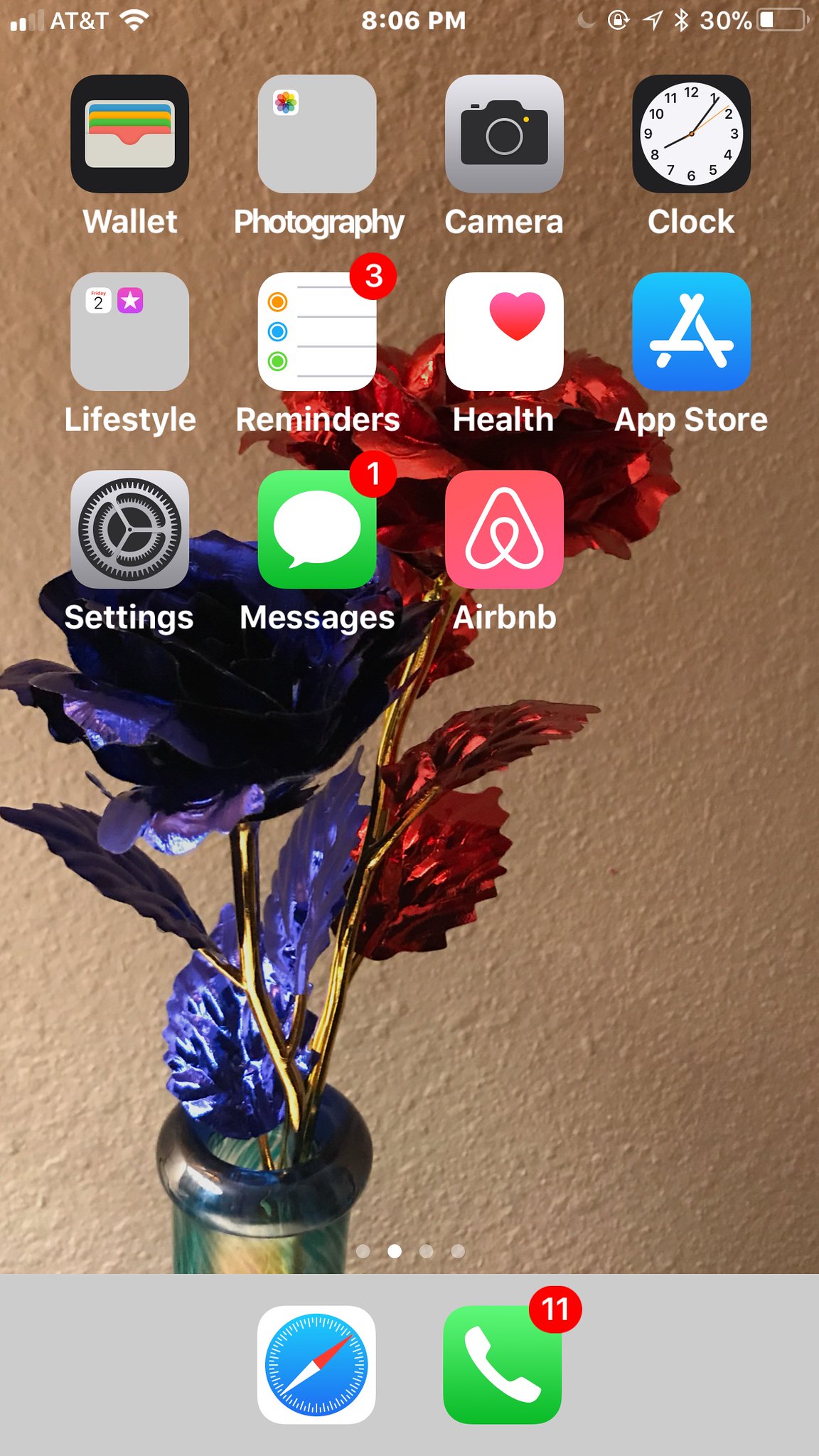The image is a screenshot of an Apple iPhone home screen. In the upper left corner, the cellular signal strength shows two out of four bars filled in white, and next to it, light white text reads "AT&T." To the right of the carrier name, there's an icon with four circular lines stacked on top of one another, indicating Wi-Fi or connection status. About two inches to the right, the time is displayed as "8:06 PM" in white text. Further to the right, it shows "30%" for the battery level, accompanied by a battery icon that is less than half filled in white.

Below the status bar, a series of app icons are arranged in a grid. Starting from the top left, the first app is the Wallet app, followed by the Photography app, the Camera app, and the Clock app, which features a small clock image above its label. Moving to the next column, there is the Lifestyle app with a purple icon, displaying a notification badge of two in a white box. The Reminders app, marked by a red circle with the number three, follows. The Health app is next, and then the App Store, identifiable by its blue icon.

On the row beneath, we see the Settings app, the Messages app with a red notification badge showing the number one, and the Airbnb app. The phone's background image is a visually appealing red and purple plant set in a thin pot.

Along the bottom dock, there are additional app icons, starting with the green Phone app, which has a red notification badge with the number eleven.

Overall, the layout is typical for an organized iPhone home screen, featuring a mixture of functional and lifestyle apps against a vibrant, nature-inspired background.